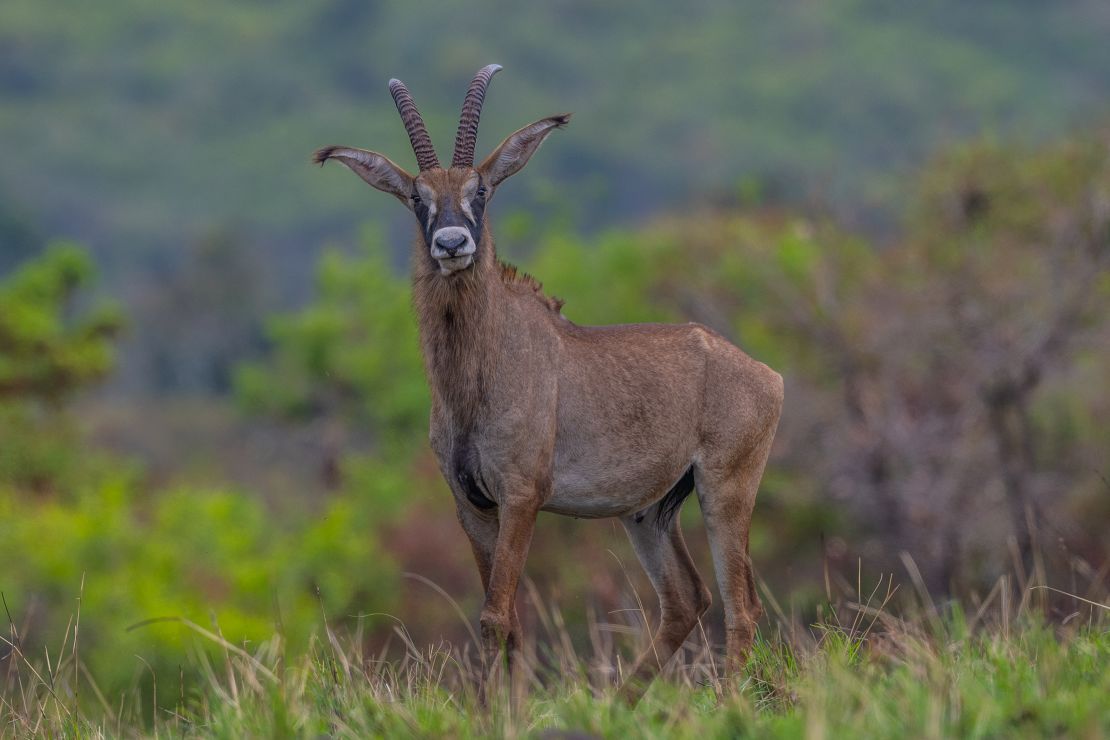In this photo, we see an animal that appears to be a cross between a deer and a goat, perhaps a gazelle. This creature stands in a field of grass, which is mostly green with some dead spots, indicating it may have been grazing there. The animal features brownish-reddish fur and has distinct black and white markings around its nose and mouth, with a particularly dark snout. Two cylindrical horns extend from its head, curving slightly backward, and it boasts long, pointy ears that stick up and out. The animal has a noticeable mohawk-like strip of hair standing up along its neck to its upper back. It is positioned sideways but looks directly at the camera, appearing keenly aware of being photographed. The background is very blurry, showcasing a hint of mountainous terrain and trees, focusing all attention on the animal. The ground around it is dotted with weeds and grass, making it clear that the animal is the central and only significant subject in the image.